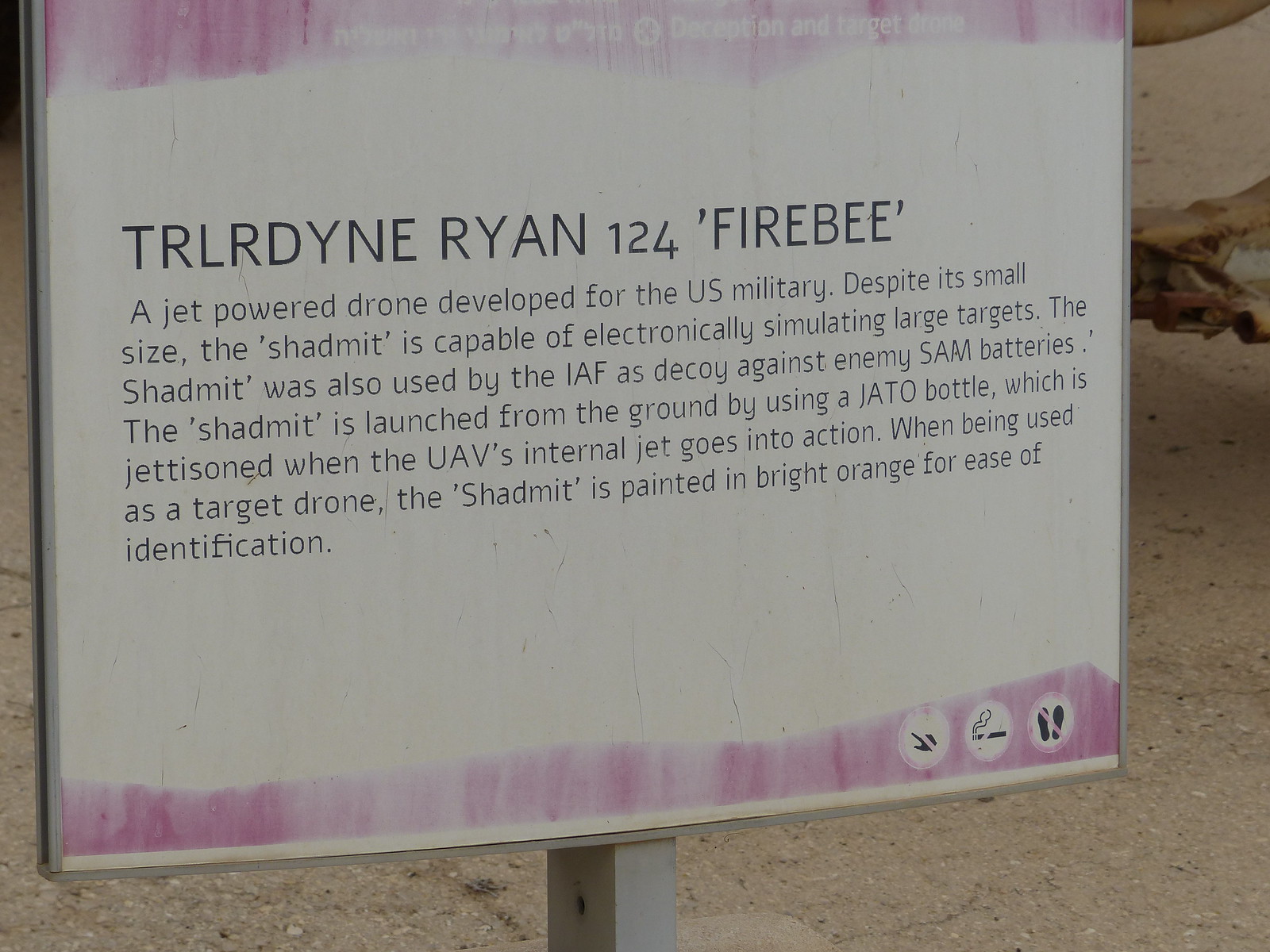This outdoor informational sign dominates the photograph and appears to be for a display not visible in the image. The sign features large black lettering at the top stating "TRLRDYNERYAN124 'FIREBEE'." Below that, in smaller text, it describes a jet-powered drone developed for the U.S. military. Despite its small size, the "Shadmint" is capable of electronically simulating large targets and has been used by the IAF as a decoy against enemy SAM batteries. The Shadmint is launched from the ground using a JATO bottle, which is jettisoned once the UAV's internal jet activates. When used as a target drone, it is painted bright orange for ease of identification. The lettering is black on a white background with a purple-pink border on the top and bottom of the sign. Additionally, there are small graphical images in the lower right of the sign indicating no touching, no smoking, and no walking. The ground below the sign appears sandy and gravelly.